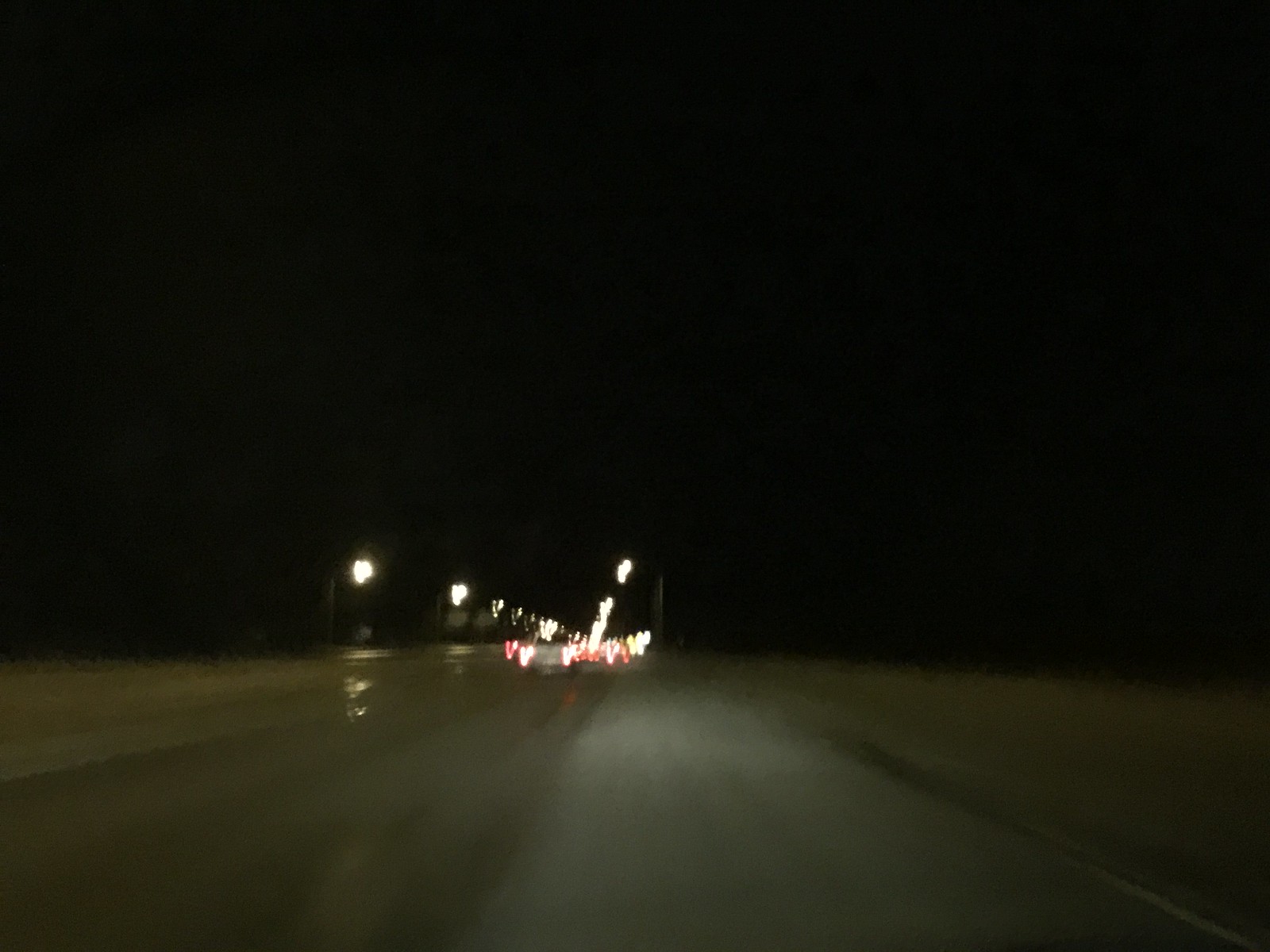In this blurry nighttime photograph, the top half is dominated by a pitch-black sky, creating a stark contrast with the lighter gray road that occupies the bottom half. The road stretches into the distance, converging to a point at the center of the image's background. Faint white dots, possibly streetlights, punctuate the upper area of the scene, with subtle, vertical lines suggesting the poles that support them. Additionally, a few distant cars are visible, indicated by their red and white brake lights, which blend into the haze and add a sense of depth to the composition. The overall blurriness gives the scene an abstract, almost dream-like quality.